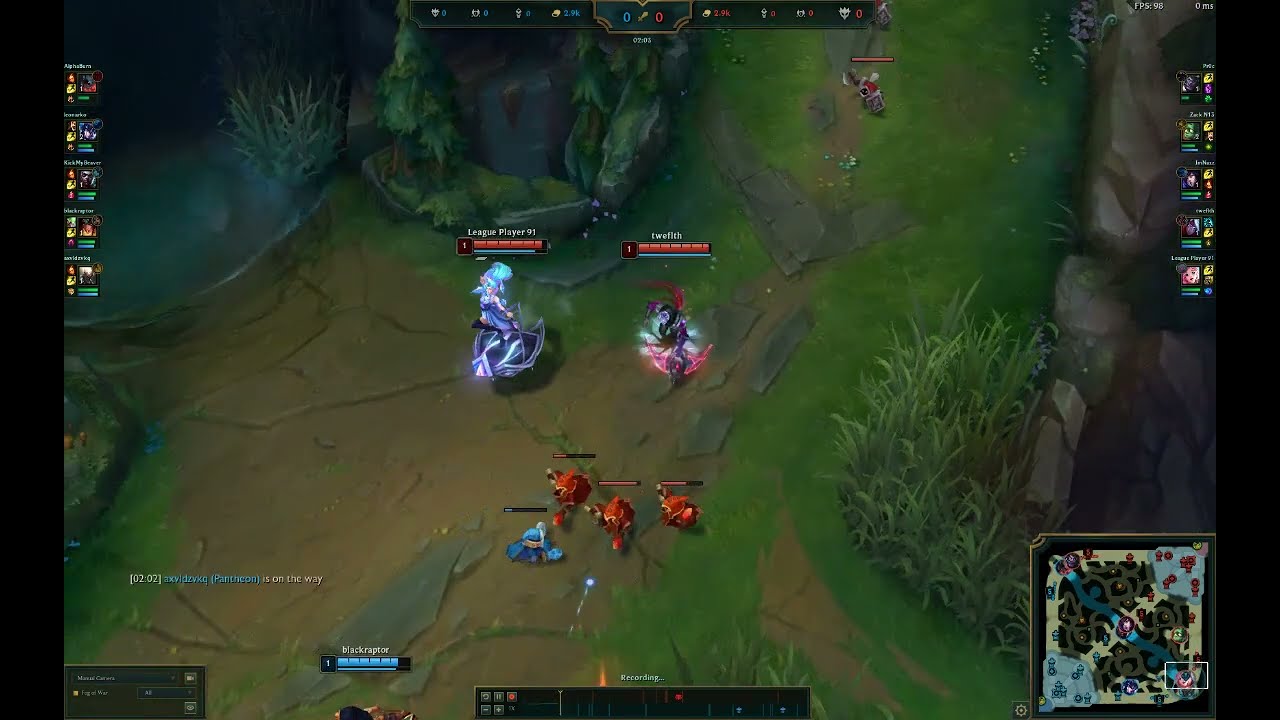The image is a screenshot from a video game, most likely "League of Legends" based on its interface and elements. The view is aerial, capturing a bit of land featuring a pond, grass, and clusters of pine trees. Central to the image are two characters standing next to each other, each with red health bars above their heads and yellow text nearby. Surrounding them are smaller creatures with their own health bars, suggesting an ongoing battle.

At the bottom of the screen, a recording indicator is visible, alongside various interactive elements like a chat box in the bottom left displaying messages such as "something is on the way" and a username. Icons of other players involved in the game are aligned along the left side of the image. On the right, the scene includes more grass and a path lined with rocks, populated by five visible enemies, hinting at a combat situation.

In the bottom right corner, a mini-map shows the characters' locations within the game world, while the upper part of the screen features a score bar set at zero to zero, possibly indicating the start of a match. The black and dark grey panels along the bottom display additional game information and controls. Overall, the scene is rich with interactive elements and hints at an action-packed moment in the game.